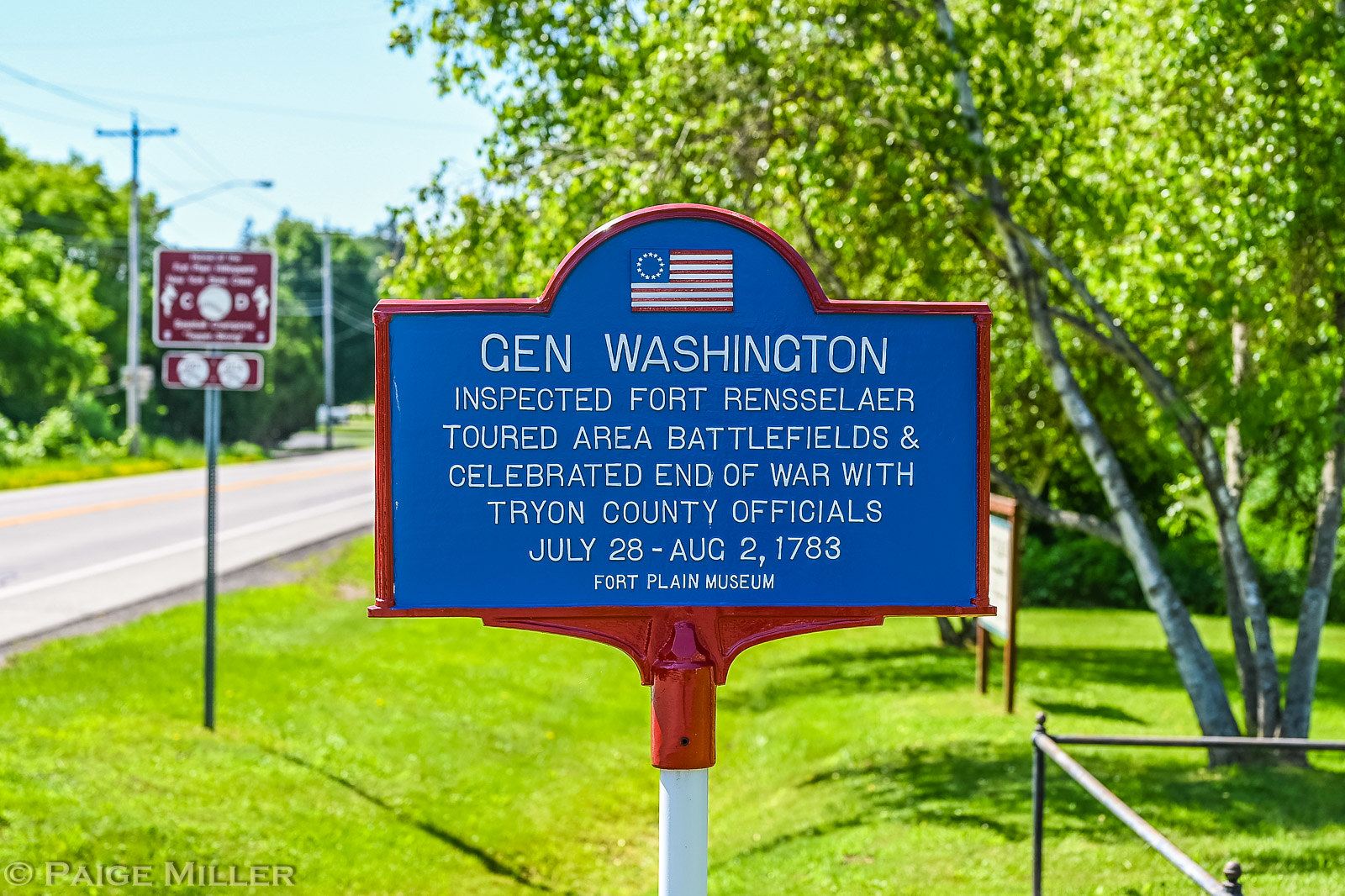In this brightly lit outdoor scene, a detailed image captures a lush, expansive grassy field. At the bottom right, a wooden fence outlines the area, while numerous trees populate the top right corner. On the left side of the image, a well-maintained single-lane road, accompanied by streetlights and electrical poles, enhances the setting. The sky is a brilliant blue, and the entire scene is bathed in bright sunshine, emphasizing the day time of capture.

Central to the image is a prominent sign mounted on a white pole. The sign has a distinct design: a red frame with a blue background in the middle. The top part of the sign features an American flag with a circle of ten stars. The white text on the sign reads: 

"General Washington inspected Fort Rensselaer, toured area battlefields, and celebrated end of war with Tryon County officials. July 28th to August 2nd, 1783, Fort Plain Museum."

Further back behind the main sign, another banner can be seen but is not legible. Additionally, there is a maroon sign with white text and a two-part design: a square at the top and a rectangle below, both bordered in white and featuring two circles. The scene captures a mix of natural and man-made elements, blending them into a historical setting, with the overall composition emphasizing the harmonious outdoor environment. The bottom left corner of the image credits the photographer, Paige Miller.